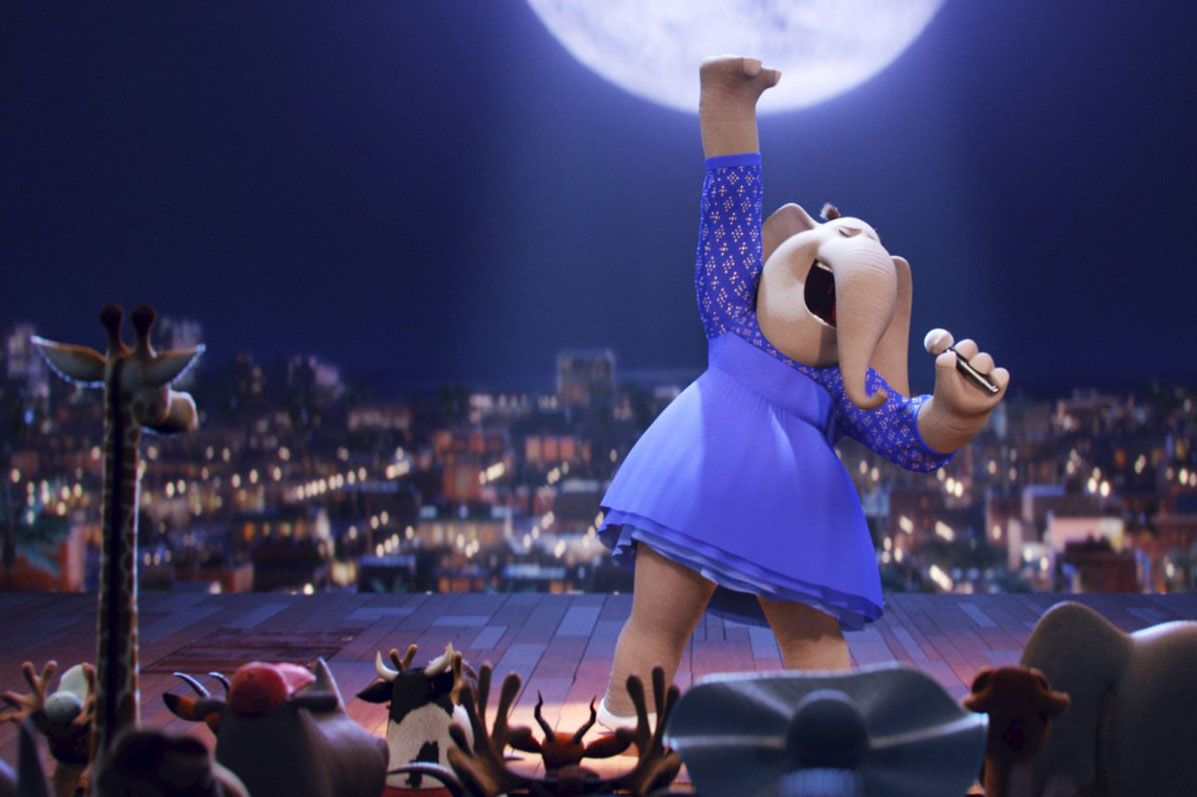This vibrant and detailed scene is a still from the animated movie "Sing," depicting an elephant girl passionately singing into a microphone on a rooftop stage. The elephant, clothed in a dazzling blue dress, stands with one hand held high and the other gripping the microphone, her mouth wide open and eyes closed, fully immersed in her performance. The backdrop features a dark blue night sky adorned with a giant glowing moon and a twinkling cityscape with blurred lights. Below her on the stage, which has a mix of red and gray tiles and wooden planks, a rich carpet lies to her left. In the audience, a variety of animals, including a giraffe, deer, cow, and possibly a hippopotamus, are visible from behind, all dressed in attire, adding to the lively atmosphere. The scene is further illuminated by a spotlight focused on the singing elephant, highlighting her as the star of the show.